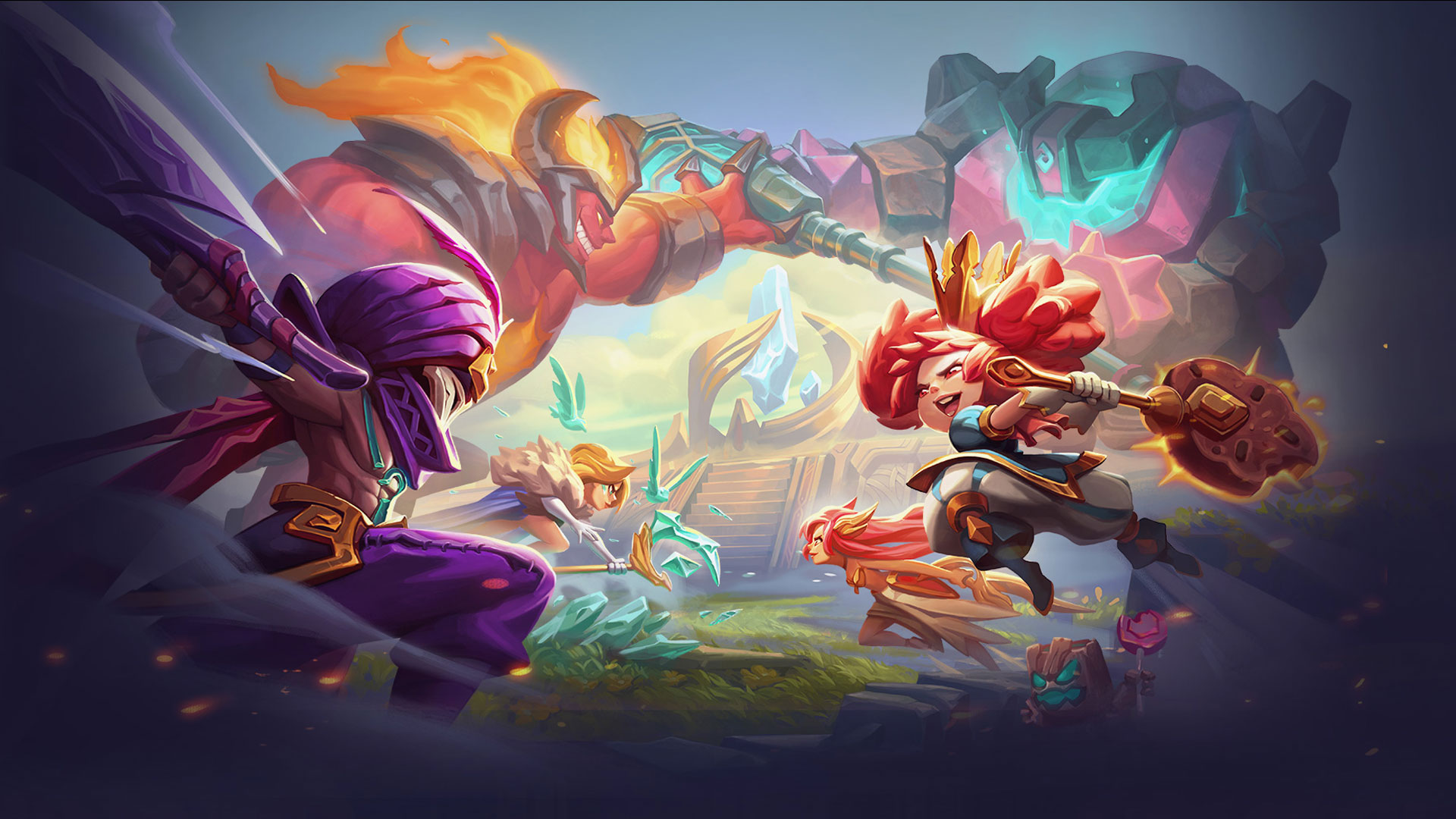The vertically aligned rectangular cartoon image depicts an intense scene, possibly from a kid's animation or video game. The background transitions from light gray-blue at the top to dark black-gray at the bottom and left side. Dominating the scene, two large, faded beasts appear in the background: the one on the left has flame-like yellow hair, devil horns, a big smile, a red face, and bulging red arms, while the other at the top right is a giant robot with a singular eye in the middle of its green and pink bolted frame. 

In the foreground, four detailed characters stand out. On the left, a shirtless purple-clad genie with a turban and puffy pants carries a sword. To the right, a girl with enormous puffy red hair holds a large hammer or club with an irregularly shaped metal top. Behind them, two more female figures are visible: one with gold hair wielding a gold weapon, and the other with long flowing red hair.

The middle section of the image bursts with color, featuring golden metal leaves forming a near-circle, green rocks, and possibly a green flying bird. The bottom contains a glowing bluish-green mythical creature, and gold steps lead up to a spiraling gold structure with a diamond-like object at its center.